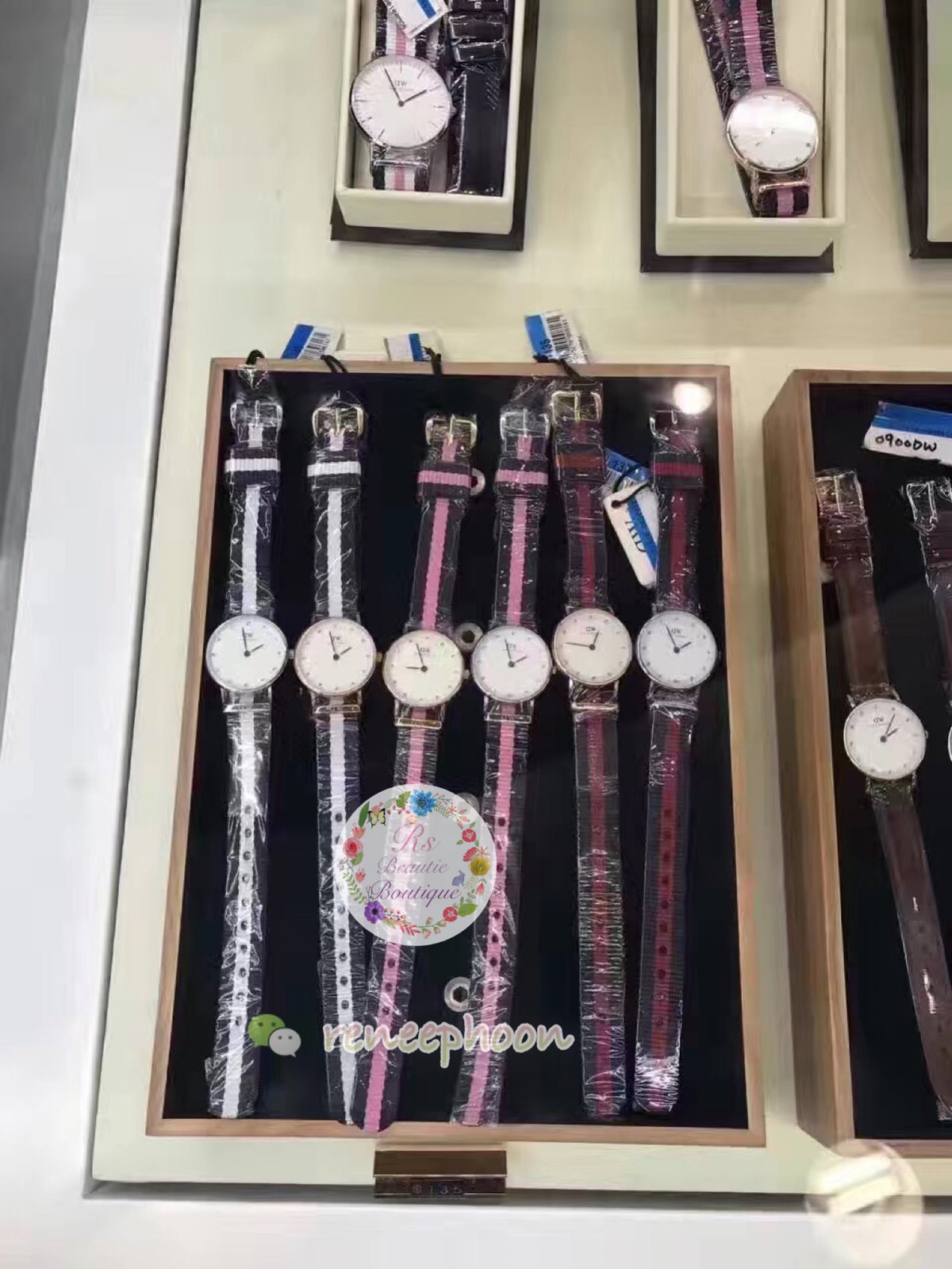The image depicts a meticulously arranged display of wristwatches, each nestled within its own rectangular wooden compartment. The compartments are lined with a rich black suede that provides a sumptuous backdrop, enhancing the elegance of the collection. Each watch features a pristine white face, creating a stark contrast to the varying colors and styles of the bands.

The bands themselves exhibit a rich variety of hues: some are a delicate pink, others a deep, regal purple, while some are pure white or shades of brown. The craftsmanship of the bands is highlighted by their leather texture, with visible lines and grains accentuating their authenticity. The watches are all encased in a transparent, presumably plastic, covering that protects them while allowing their intricate details to shine through clearly.

This sophisticated arrangement suggests the setting of a high-end jewelry shop, where meticulous attention to detail and quality presentation are paramount.